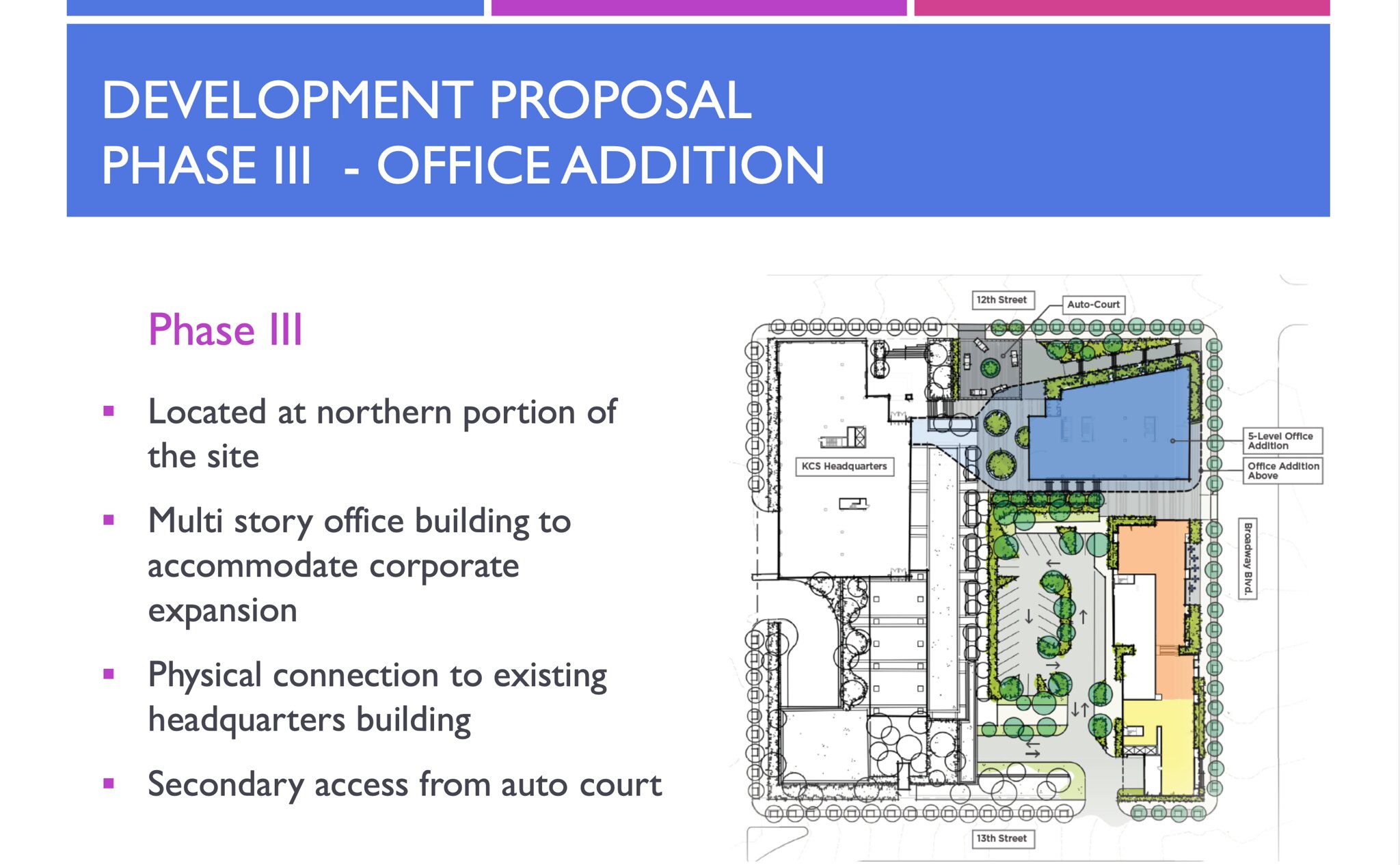The image is a scanned PowerPoint slide displaying a detailed Development Proposal for Phase 3: Office Addition. At the top, a blue header with white text reads "Development Proposal Phase 3: Office Addition." Below, a purple rectangle prominently featuring "Phase 3" in pink letters introduces a series of key details. The proposal outlines a multi-story office building, located at the northern portion of the site, intended to accommodate corporate expansion. Key features include a physical connection to the existing headquarters building and a secondary access point from the auto court. To the right, a colorful floor plan depicts the new additions, annotated with arrows and text boxes for clarity. The map displays green areas symbolizing shrubs or trees, along with labels such as "Broadway Boulevard," all set against a white background.